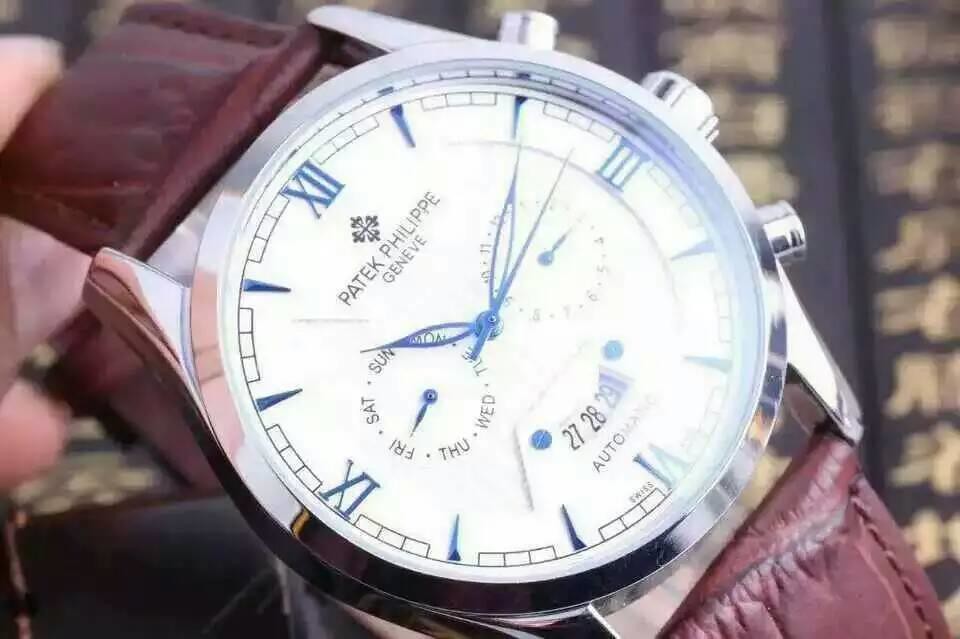A detailed close-up photograph of an elegant men's wristwatch crafted by Patek Philippe. The watch features a stainless steel case with three intricately designed knobs on the side, each serving a unique function. Prominently displayed on the face are the inscriptions "Patek Philippe" and "Geneve," symbolizing the brand's prestigious heritage. The dial showcases black Roman numerals that add a touch of classic sophistication, while the hour and minute hands are slender, delicate, and shaped like elongated teardrops or leaves, crafted in a fragile-looking black wire. The black slender second hand resembles a needle, sweeping gracefully across the dial.

Flanking the central hands are two sub-dials; the left one displays the days of the week with a tiny hand currently pointing to Friday, and the right one shows a date wheel marked by another slim hand. At the bottom of the watch face, a separate window reveals the current date, indicating the 28th with visible numbers 27, 28, and 29.

The watch is secured by a well-worn, reddish-brown leather band that exudes a vintage charm. The attachment points of the band show signs of use, adding character and history to the timepiece. The leather band is stitched with thread matching its color, giving it a cohesive and refined appearance.